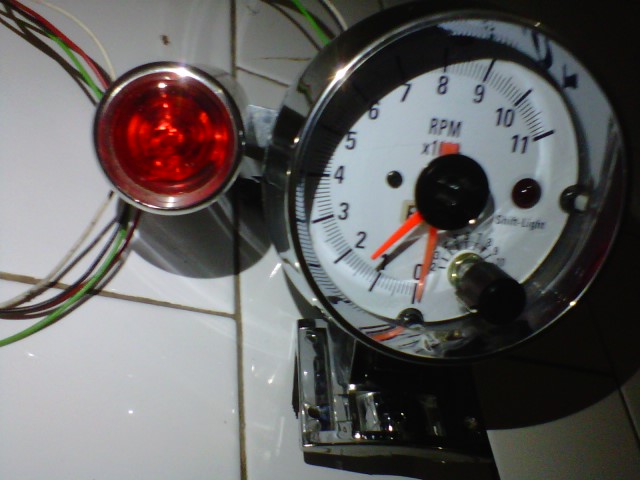The photograph showcases an RPM meter with a classic dial design, situated against a white tiled surface, which could either be a floor or a table. The white tiles are separated by gray grouting and occupy the left side of the image. A distinctive red light with a chrome encasement is also visible on this side. Extending from the 10 o'clock to the 8 o'clock position on the meter are a series of red, black, and green wires, trailing off the left edge of the frame.

The RPM meter's right side, still positioned atop the white tiles, features a darker strip of background running vertically along the image's edge. The dial is encased in a chrome housing unit, with an additional square piece of chrome or steel at its base, which may or may not be secured to the tile surface.

The face of the RPM meter is white, with orange dials set against the clean background. The numerals begin at 0 at the bottom center and increment clockwise, reaching 11 at the 2 o'clock position. The overall arrangement suggests a meticulous and potentially operational setup, despite the ambiguity of its connectivity.